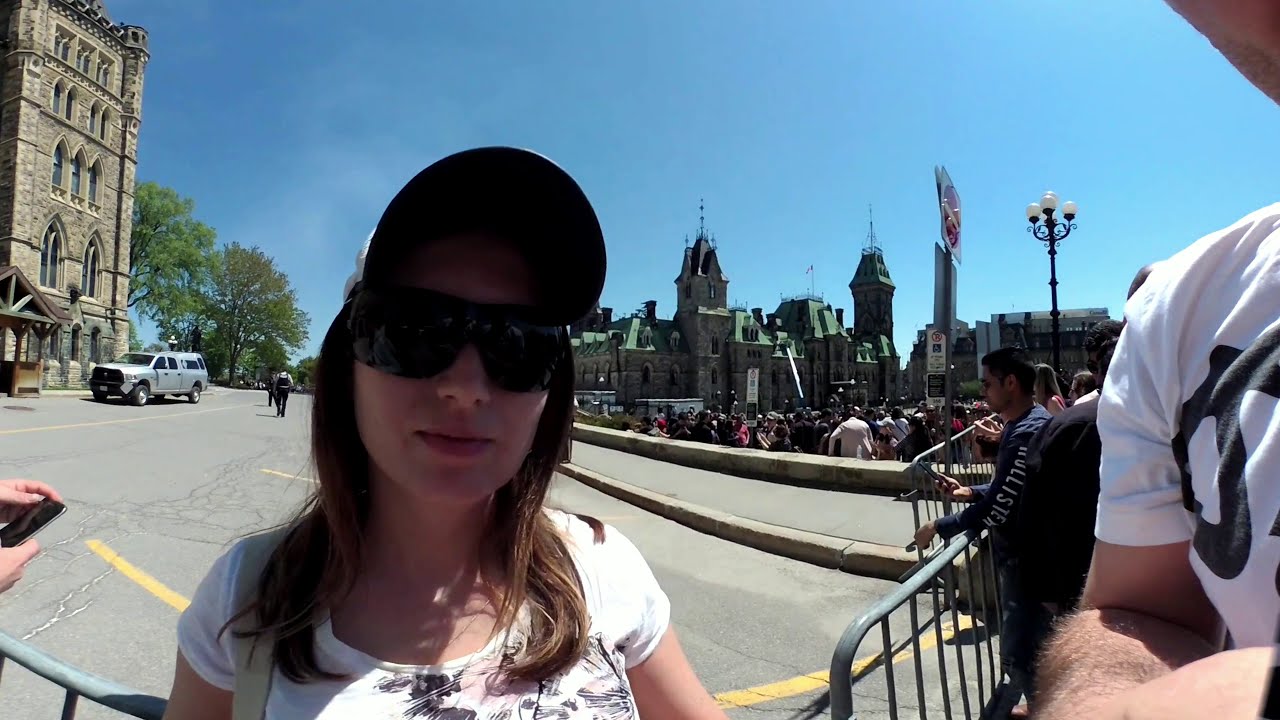The image captures a lively street scene centered around a young Caucasian woman. Positioned slightly to the left of center, she gazes directly at the camera with a possible hint of taking a selfie. She sports large, dark sunglasses and a black hat over her light brown hair, which flows just past her shoulders. Her white shirt, adorned with black designs, and the strap of a purse resting on her right shoulder, are clearly visible. The photograph frames her from the chest up, and she is set against a busy backdrop.

To the right of the frame, a man's arm clad in a white and gray T-shirt extends into the shot, perhaps holding a phone or camera. He's partially visible, with hints of his face showing at the top of the image and his arm extending downwards. Behind him, a guardrail traces the scene, beyond which clusters a densely packed crowd of people.

In the distance behind the woman, on the left, architectural details suggest the corner of an old church with light brown arched windows. A truck is parked nearby, and a small figure that resembles a security guard stands near the building. Additionally, trees and what look like newer constructions designed to mimic castle-like structures are also observable in the background. The sky overhead is a clear, bright blue, free of clouds, enhancing the vividness of the scene. Yellow lines marking parking spaces and directional lines on the street indicate a well-defined roadway curving off towards the two o'clock direction. The atmosphere is bustling, with people leaning against rails and moving along the street, reflecting a vibrant outdoor setting.